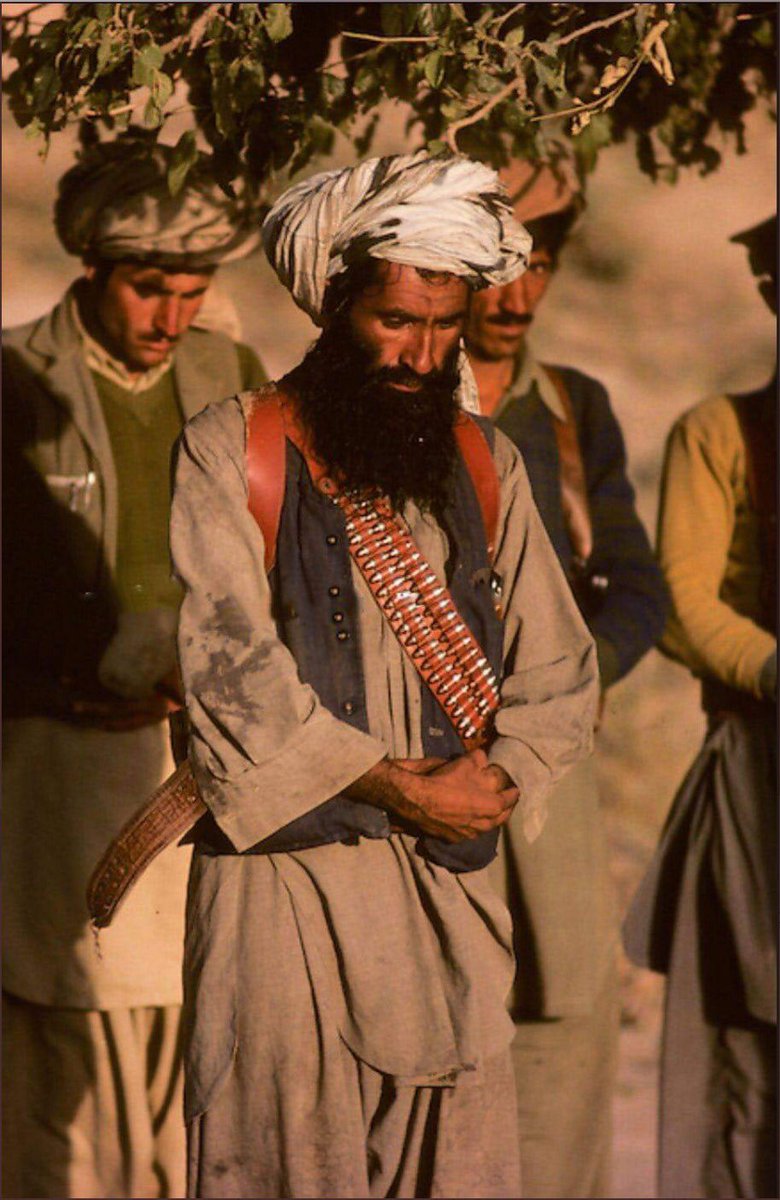In this image, we see a group of men, appearing to be of Middle Eastern descent, with their heads bowed, exuding a serious and contemplative mood. The central figure, with a full black beard, dons a gray robe and vest, and wears a white turban. Draped across his shoulder is a striking red and white bullet band. To his left stands another individual in a green shirt and gray vest, also looking downward, and wearing a tan turban. On the right, a man with a green and blue shirt looks directly at the camera, while only the arm of a fourth individual in a yellow shirt is visible. The blurred background features light brown tones and the hanging leaves of a green plant, suggesting the image might have been taken in a desert setting.